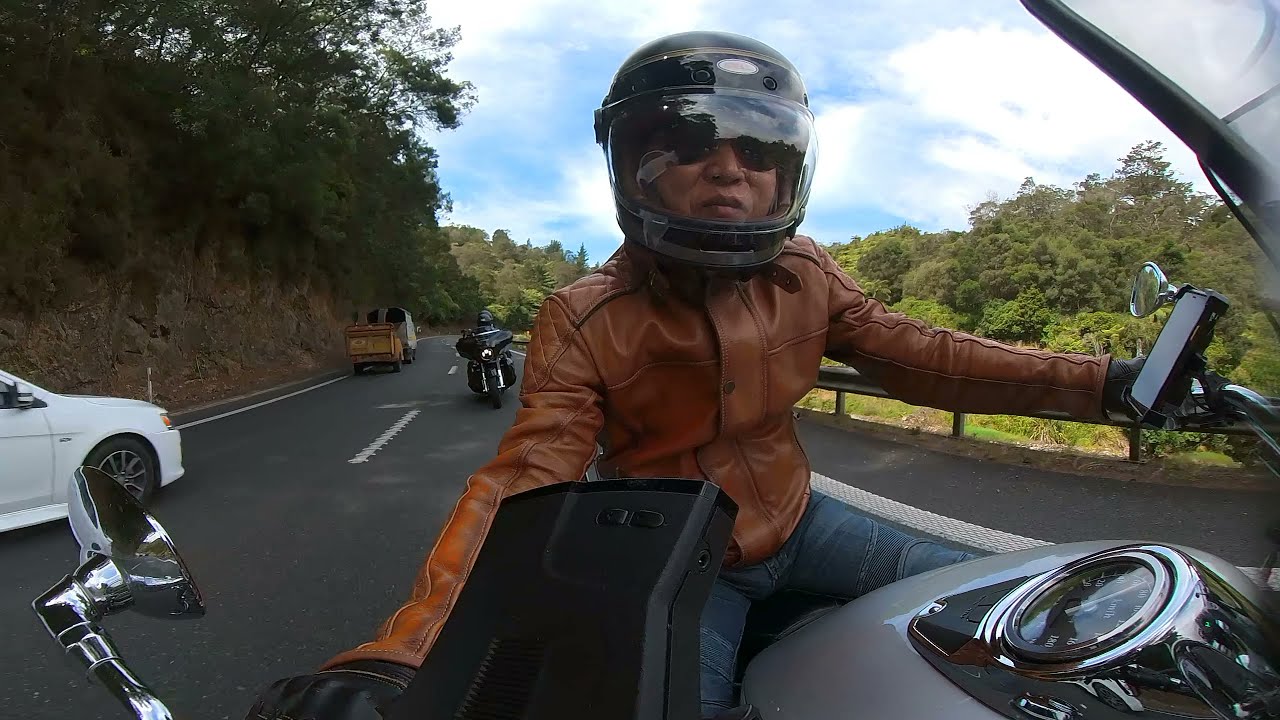This detailed photograph captures a motorcyclist riding down a winding, two-lane road cutting through a cliffside with a scenic guardrail and lush greenery. The image is taken from a fisheye or 360-degree angle from behind the motorcyclist, giving a dramatic rear-view perspective as if the camera is mounted on the handlebars. The motorcyclist is dressed in blue jeans, a brown leather jacket, and a dark helmet with a clear visor pulled down over sunglasses. You can see their hands gripping the handlebars, which are equipped with a directional GPS device. A silver motorcycle with chrome accents is partially visible, conveying the sleekness of the ride. Behind him, another motorcyclist on a black motorcycle follows closely. On the road, a white car, possibly a van towing a small luggage compartment, travels in the opposite direction. The left side of the frame features a steep dirt hill with trees, while the right side shows a lower guardrail with more greenery. The sky is a vivid blue, dotted with fluffy white clouds, making for a picturesque and adventurous scene.